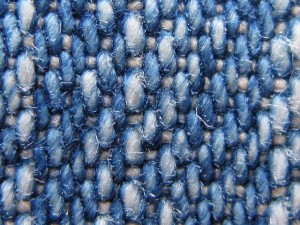This image is an extreme close-up of a swatch of fabric, potentially from a blanket or sweatshirt, showcasing a detailed woven or knitted structure. The predominant color scheme is blue, with threads in dark blue, light blue, and white. Along the right-hand border, the stitches are uniformly white. The threads are visible in various sizes and shapes, predominantly oblong and rice-like, with some being narrow at the top and wider at the bottom. Smaller, almost square-shaped white threads crisscross through the fabric in the opposite direction. The intricate threading spans the entire image vertically, with bits of thread escaping from the knots and stitches, highlighting the fabric's textured and intricate design.